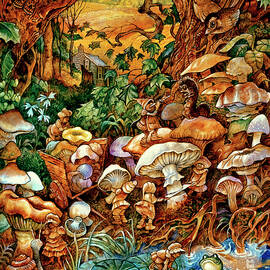The image portrays a whimsical, fantasy scene of a densely packed mushroom grove, intricately drawn or digitally rendered in a square format. The mushrooms, in a harmonious blend of colors such as dark brown, light brown, cream, and dark orange, populate the foreground, while little gnomes or fairies busily harvest them. Some creatures are cutting the stems, and others are carrying mushrooms towards a modest, tiny wooden cart filled with more mushrooms. One figure is placing a mushroom onto the cart, where another is diligently arranging them. 

In the bottom corners, a green frog can be seen near a blue patch of water, accompanied by a green lily pad at the bottom center. The background reveals a lush forest area with greenery and trailing leaves climbing up the trees, complementing the scene with bursts of green on the left side. The sky above is painted in deep yellow with tinges of orange and clouds, transitioning to an orange-yellow hue at the top center. Near the top right, two birds gaze down at the gnomes from their perch.

Further in the distance, a small house or cabin sits, nestled among more green grass dotted with small white flowers. The gnomes, with their pointy hats, long tunic-style shirts, tights, and little boots, add a charming touch to the image, which maintains a palette of browns, greens, yellows, and oranges. The overall composition captures an enchanting and detailed woodland scene teeming with life and activity.